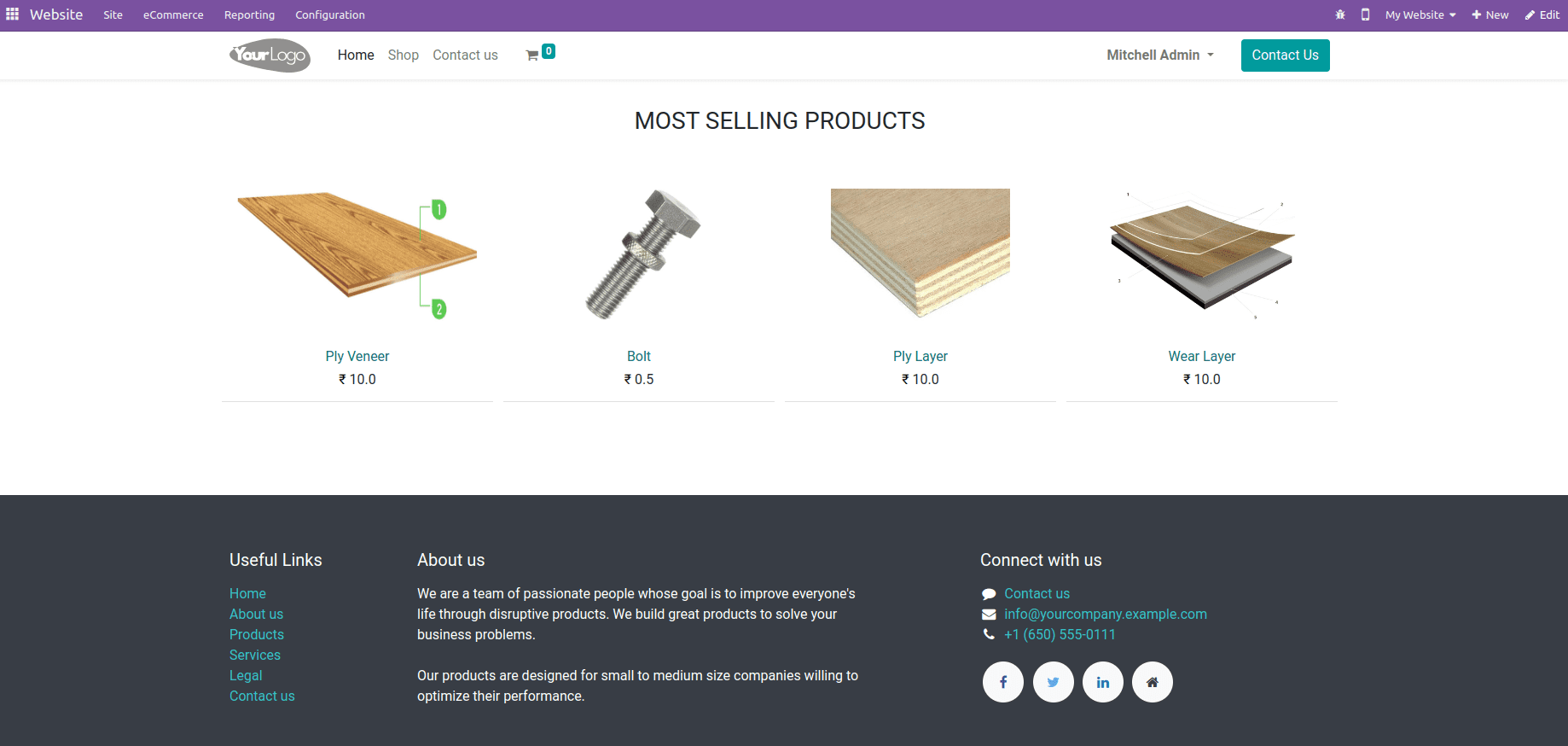This image is a detailed screenshot of an e-commerce website template. The header graphic at the very top is a bold purple color, indicating key components of the website. In the upper left-hand corner, instead of a company name, it reads "website" followed by sections labeled "site," "e-commerce," "reporting," and "configuration." Directly below is a designated area for the user's logo.

The primary background of the page is white. Centrally located on the page is a heading that reads "Most Selling Products," showcasing four example products. The first product appears to be a piece of plywood labeled "Ply Veneer." Adjacent to it is a large image of a bolt with the straightforward label "Bolt." Next is a close-up of a plywood stack named "Ply Layer," and on the far right, there is a piece of wood possibly topped with laminated tile, labeled "Wear Layer."

At the bottom of the image, the footer is a muted gray. The footer section is organized into three primary areas: "Useful Links" on the left, "About Us" in the center, and "Contact / Connect with Us" on the right, indicating where the user can input relevant information for a complete website experience. This template provides placeholders and a structured layout, offering a clear visualization of a functional e-commerce website.